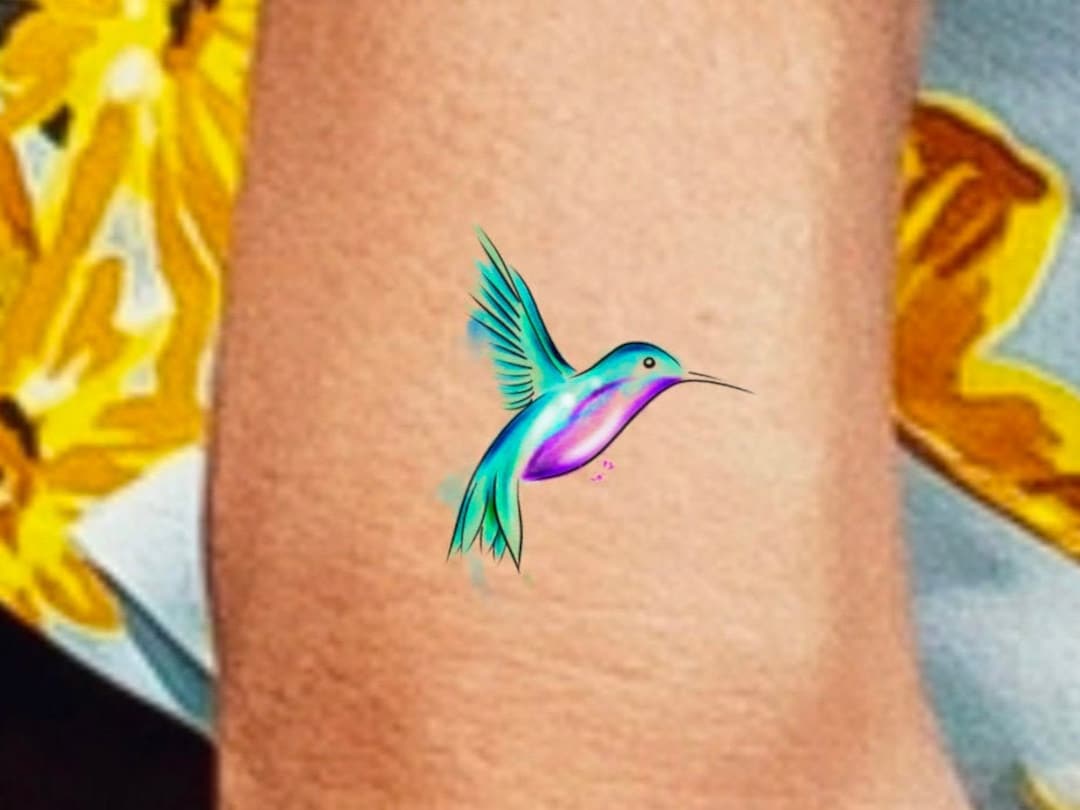A pristine white towel adorned with large, vibrant yellow and brown flowers serves as the background. Beneath it lies a sturdy brown table. In the foreground, there's a person's arm, recently tattooed with a delicate and beautifully detailed hummingbird. The hummingbird boasts a sharp, elongated beak and a small, black eye. Its underside is painted a lovely shade of purple with touches of white, while its upper body transitions into hues of green and dark blue. The bird's wings, poised mid-flight, glisten with a blend of green and blue feathers, capturing the essence of motion and grace.